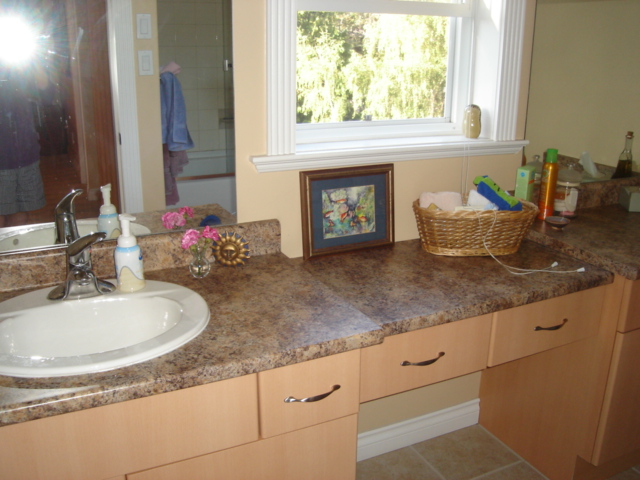This photograph appears to be taken in a modern washroom. The floor features a brown tile pattern accented with white grout lines. Along one wall, sleek light wood cabinets equipped with silver handles provide a stylish touch. Topping these cabinets is an expansive countertop, light brown in color adorned with darker brown decorative patterns. 

On the left side of the countertop sits a pristine white sink fitted with a silver faucet. Adjacent to the sink is a soap dispenser, a purple flower, and a decorative gold sun. Above the sink hangs a large mirror that captures the reflection of the person taking the photo, along with a noticeable camera flash. The mirror also reflects the outline of a bathtub situated behind the photographer.

Following the length of the countertop toward the right, there is a framed picture in a brown frame, a basket, and what appears to be a can of hairspray. Above this area, a white window sill with a window offers a glimpse of the outdoors, revealing verdant green trees or bushes bathed in sunlight.